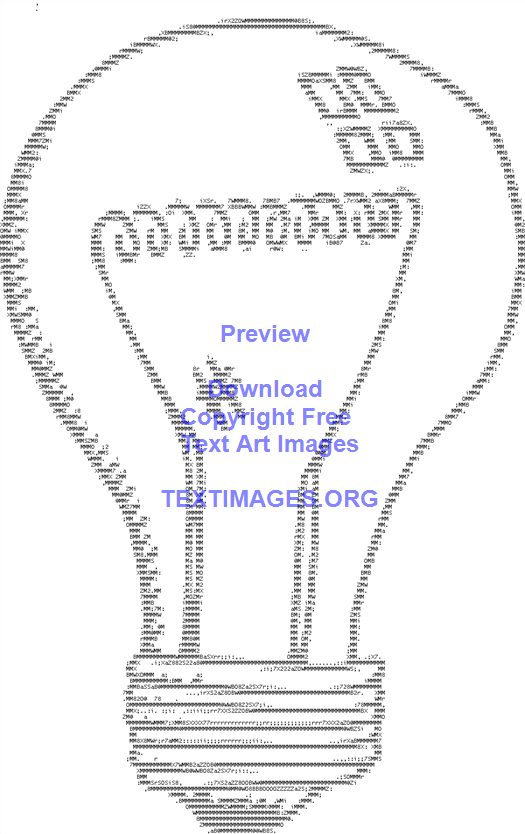This image is a detailed ASCII art illustration of a lightbulb, composed entirely of black and white text characters. The intricate design includes six distinct layers of text forming the bulb itself, with a socket at the base and ten text-formed wirings at the top, simulating the light-emitting components. The composition contains black, white, and blue text, with the center of the bulb displaying the words: "Preview, Download, Copyright Free, Text Art Images" in that order. At the bottom is the website address, textimages.org, though it appears less prominently. The overall appearance exudes a classic, vintage digital aesthetic, showcasing an old yet fascinating method of creating images via text characters.